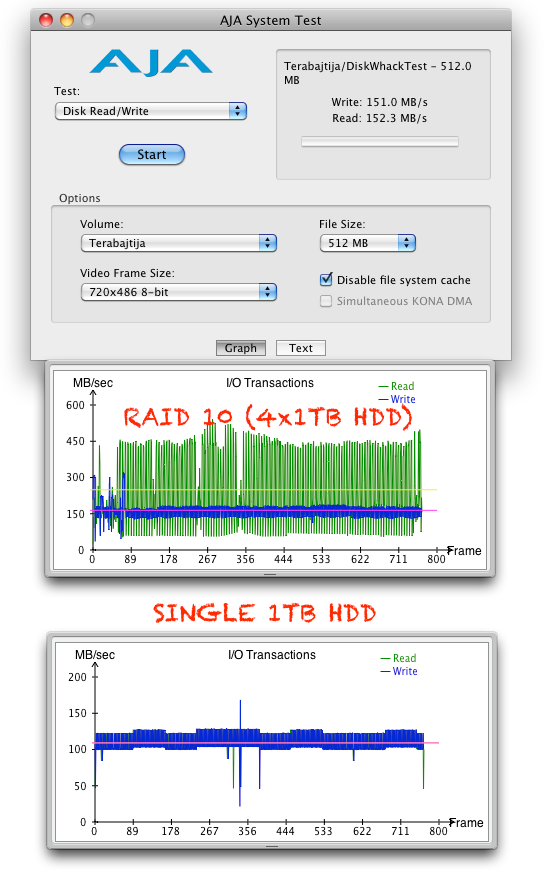The image displays a collage of screenshots, presumably captured from a Mac device, that visually detail an AJA System Test interface used for measuring disk read/write performance. At the top of the display, the main screenshot features a white background with blue text that reads "AJA System Test." To the left, three circles in red, yellow, and clear indicate GUI elements typical of Mac OS applications. Below is a light blue box labeled "Start," followed by various dropdown menus and options for selecting test parameters such as disk, read/write operations, and file sizes. These menus include terms like "Volume, Value, Frame Size, and File Size."

Beneath this top section are two distinct graphical representations. The first graph is marked by red text indicating "RAID 10 (4x1TB HDD)," with horizontal and vertical axes measuring up to 600 MB/sec and 800 frames respectively, showing green and blue lines representing read and write operations. The second graph below this features similar metrics for a "Single 1TB HDD," with axes labeled 0 to 200 MB/sec and 0 to 800 frames. Across both graphs, fluctuations in the bars reflect data transaction volumes, emphasizing performance differences between RAID 10 and single disk configurations. The color scheme throughout includes shades of white, gray, black, tan, blue, green, red, and light blue, enhancing the clarity and readability of the test results.